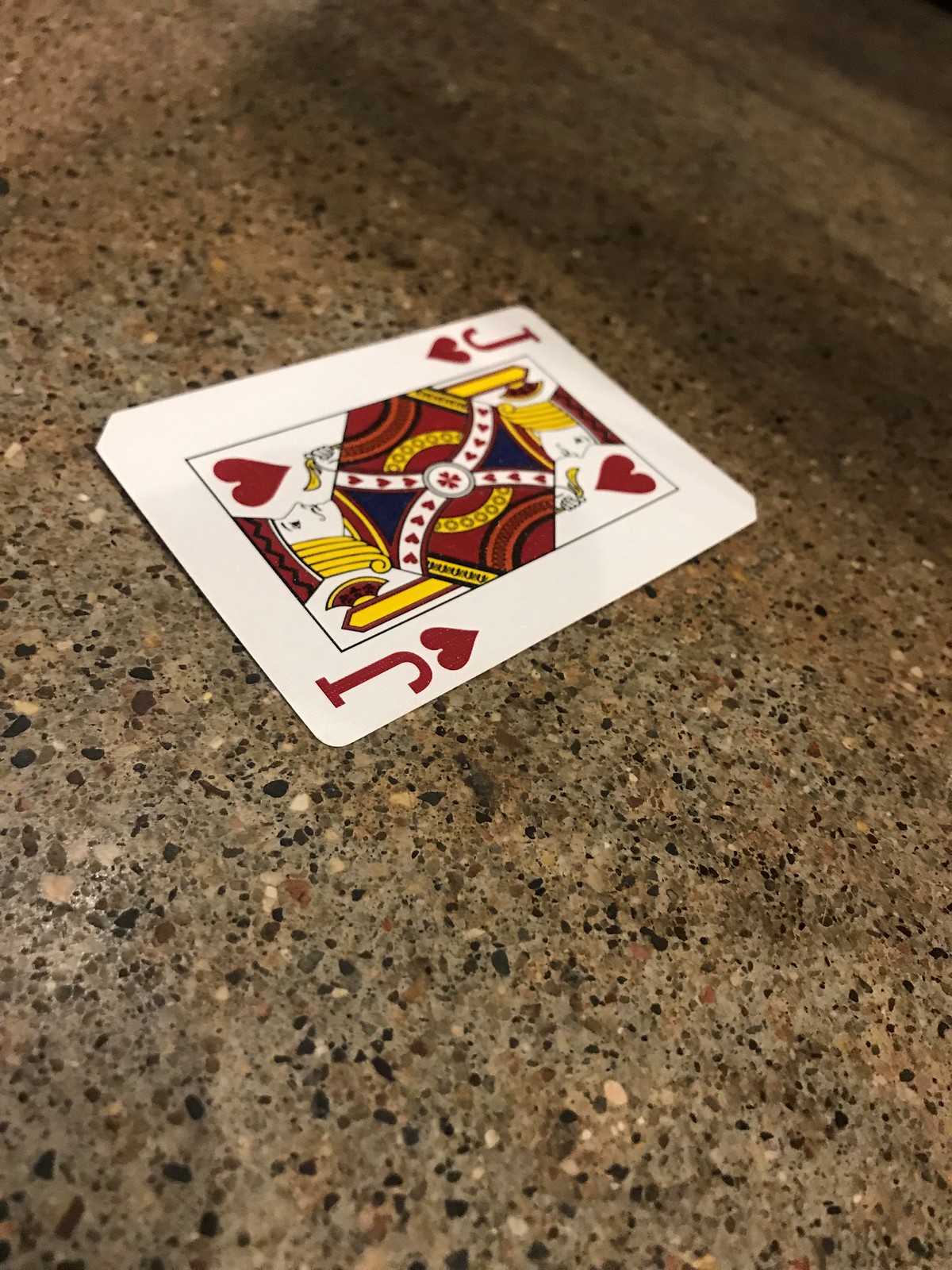This photograph features a single card from a standard playing deck, specifically the Joker of Hearts. The card itself is white with vivid red symbols. Red heart icons and a red letter "J" are prominently displayed in the upper left and bottom right corners. At the card's center, the Joker is depicted in a traditional, symmetrical design, mirrored at both the top and bottom of a vertical rectangle. 

The Joker has striking yellow hair and is shown in profile, facing towards the right side of the image. He wears a distinctive red and black hat, complementing his multi-colored attire, which includes shades of red, yellow, black, and white. In his left hand, which is raised toward his face, he holds an ambiguous yellow object, possibly the handle of a weapon or similar item.

The card is placed against a backdrop that appears to be a granite countertop, inferred from its smooth, even texture and distinctive pattern.